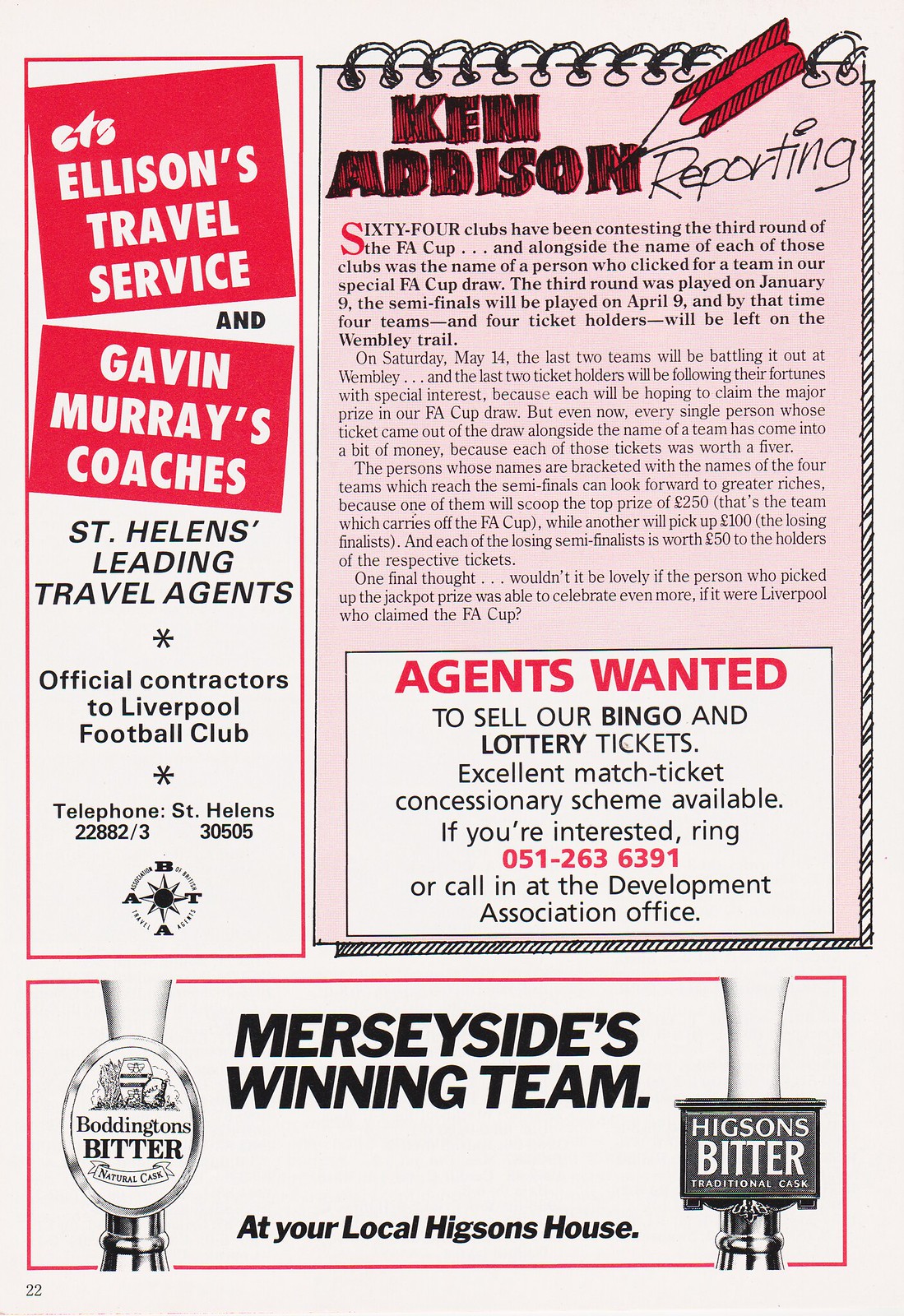The image portrays a vintage magazine page featuring a promotional section and an article titled "Ken Addison Reporting." On the left side, there are a series of red squares with white text, including "Allison's Travel Service" and "Gravenmarren's Coaches." Below these, in black font, "St. Helen's Leading Travel Agents" is printed, followed by "Official Contractors to Liverpool Football Club" separated by stars. Further down, the contact number "St. Helen's, 22882, 4-3, 30505" is displayed. The right column is dominated by the article, which discusses 64 clubs contesting in the third round of a cup, possibly the FA Cup. A hand-drawn notepad and pencil add a whimsical touch to the layout. Beneath the article, the text "Agents wanted to sell our bingo and lottery tickets" is prominently featured. The overall design showcases a mix of colors, including tan, red, white, black, gray, and pink, contributing to its old-school sports magazine aesthetic.